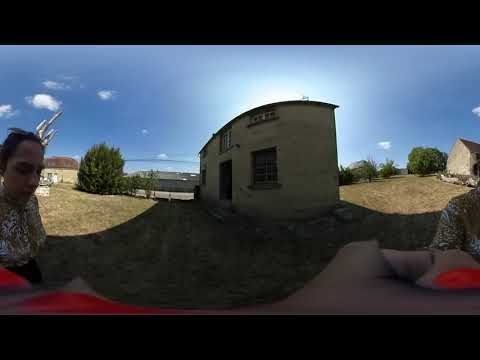In the photograph, a woman with dark hair wearing a white flowered shirt and black bottoms is taking a selfie using a 360-degree camera, resulting in a distorted fisheye effect. She is visible on both the left and right sides of the image, with her arm stretching unnaturally from the bottom left corner to the bottom right, where her fingers, adorned with red nail polish, seem to clutch the selfie stick. The central focus of the panoramic image is an old, somewhat unkempt, two-story stone or brick building, partially obscured by shadows cast by the surrounding sunlight. This building is flanked by patches of brown, earth-like ground, with hints of green vegetation, possibly indicating dirt with sparse grass. In the background, additional structures and large bushes or small trees are visible. The sky above is blue with a few scattered clouds, and the glare of the sun creates pronounced shadows, adding depth and dimension to the scene. This setting, reminiscent of a historical park or a quaint area outside the United States, combines the appearances of aged architecture and natural elements.